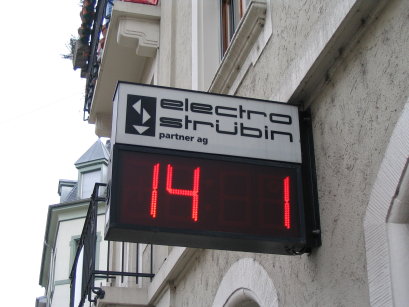This image features a sign attached to the exterior of a multi-story stucco building. The structure includes several balconies with black railings and a visible window situated above the sign. The sign itself is square in shape with a distinct logo at the top portion, rendered in black and white. The text on the sign reads "Electro Struben Partner AG." Directly beneath this text is a black box showcasing white triangles pointing in various directions. Below this graphic element is a red digital display that reads "14 1", which likely indicates the time as 1:01.